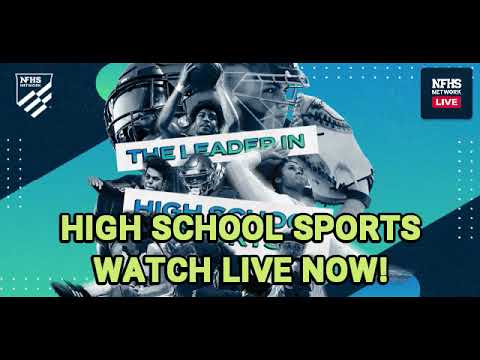The image features a vibrant collage of various high school sports players and objects, centrally condensed in a grayish to light blue hue. Prominently displayed are athletes from diverse disciplines including basketball, football, volleyball, and gymnastics. A basketball player is positioned at the top, appearing ready to make a shot, while a football player and other sports figures are scattered throughout the center.

The backdrop includes a light blue diagonal strip running from the lower left to the upper right, flanked by dark navy blue sections. The layout is accentuated by logos and text overlays: the top left corner displays an NFHS logo with a shield, while the top right corner features a black box containing "NFHS Network Live" in bold text. The bottom center of the image showcases another text segment in green with a black outline, proclaiming "High School Sports, Watch Live Now!" with an exclamation point.

The overall setup suggests that this image is likely a screenshot from an advertisement, possibly originating from a TV station or the network's website, promoting live high school sports coverage via the NFHS Action Network.